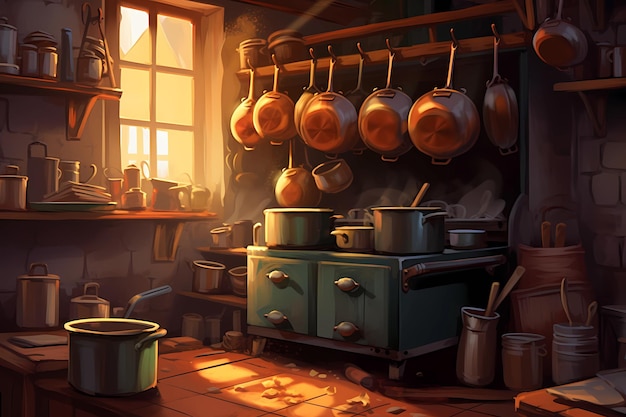This professionally rendered artwork features a detailed, old-fashioned kitchen scene dominated by a teal-grayish green stove with gray knobs. Atop the stove, several silver pots and pans are in use, some with steam rising and a wooden spoon sticking out of one. Above the stove, a large brown wooden shelf with hooks displays about a dozen shiny, brass-colored copper pans.

To the left of the stove, there's a large rectangular wooden window with amber-yellow light streaming through, casting a warm hue over the kitchen. Adjacent to the window, two sturdy wooden shelves are stocked with various containers, dishes, and pots. A wooden table with a pot sits nearby.

The kitchen's gray stone wall backgrounds the entire scene, adding to its rustic charm. The palette of the painting includes rich tones of black, white, gray, green, copper, brown, orange, and yellow, enhancing the ambiance of the old-fashioned cooking space. Every detail, from the wooden handles to the brass pans, is rendered with professional artistic skill, creating a vibrant and engaging depiction of a humble yet charming kitchen.